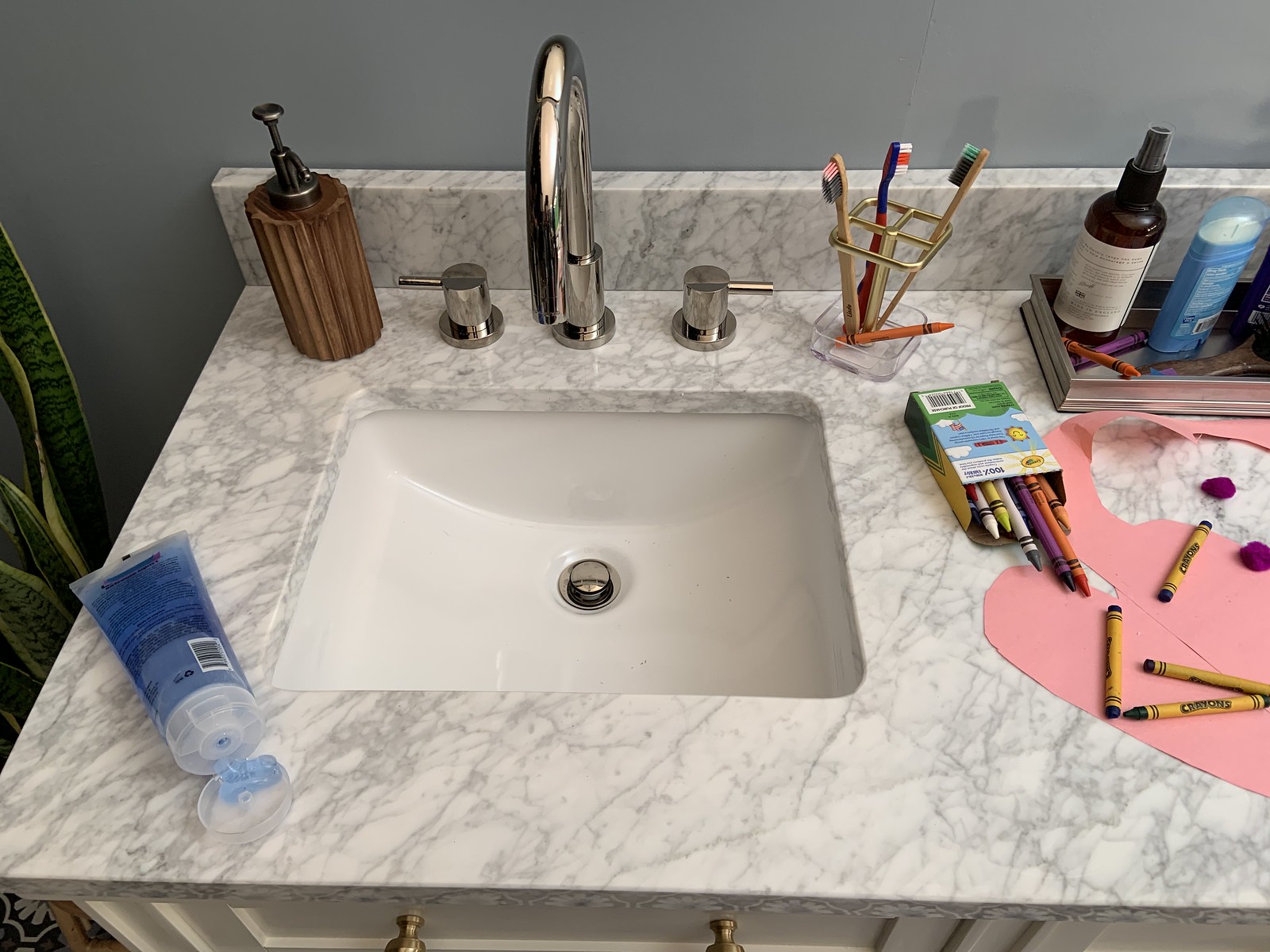In the image, a modern bathroom sink is prominently showcased against a sleek gray wall, which provides a neutral backdrop. On the right-hand side, the edge of a lush green plant is visible, adding a touch of nature to the setting. The counter surrounding the sink is a sophisticated white with grey veining, reminiscent of marble. Atop this counter is an open blue container, from which blue gel is spilling out. Nearby, there's a brown soap dispenser.

The white sink is fitted with standard chrome fixtures, including the faucet and temperature control handles. Adjacent to the sink, organized on a countertop, is a clear plastic holder featuring a gold-tipped design, which contains toothbrushes and a conspicuous orange crayon. Beneath this holder, an opened box of crayons spills its colorful contents, with some scattered onto a piece of pink paper adorned with a few purple spots.

Additionally, a silver tray rests on the counter, holding more crayons and a brown spray bottle with a white label covered in small text. Positioned to the right of this tray is a blue container, likely containing deodorant.